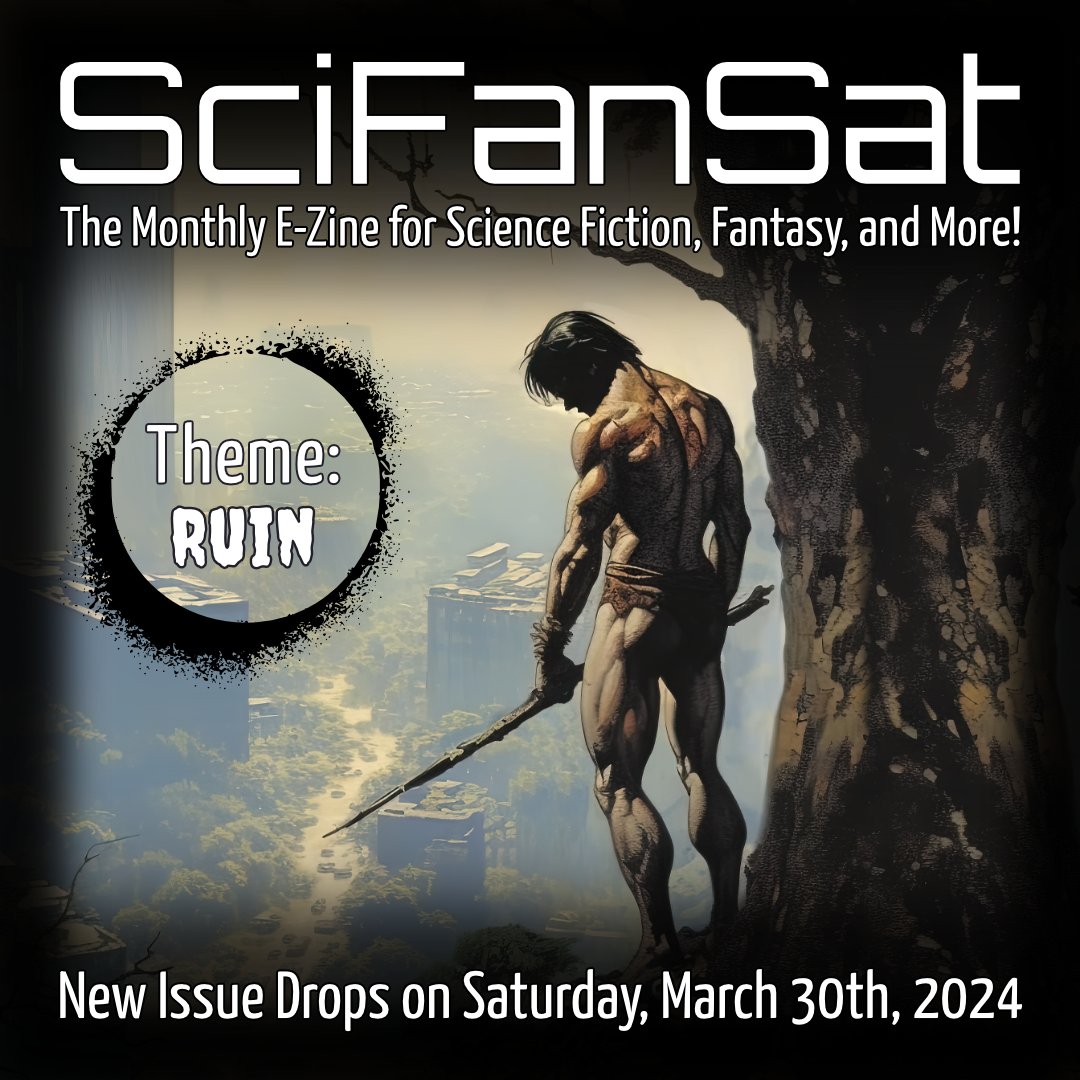This image is a detailed advertisement poster for the "Sci-Fi Fan Set," a monthly e-zine dedicated to science fiction, fantasy, and more. The top center of the poster features the title "Sci-Fi Fan Set" in bold white font, followed below by the subtitle "The monthly e-zine for science fiction, fantasy, and more." In the bottom left corner, within a nearly black circular design, the words "Theme: Ruin" are prominently displayed. At the bottom, the release date is clearly stated: "New Issue Drops on Saturday, March 30th, 2024."

Dominating the center-right of the poster is a vivid illustration of a muscular man with short black hair standing at a high elevation, looking over a ruined city overtaken by vegetation. He is almost entirely naked except for a loincloth and has wraps around his wrists. He holds a sword in both hands and gazes downward toward the overgrown city, where abandoned vehicles are visible among the reclamation. To his right stands a large tree with a dark brown trunk. The man’s face is obscured, adding a sense of mystery to the apocalyptic scene.